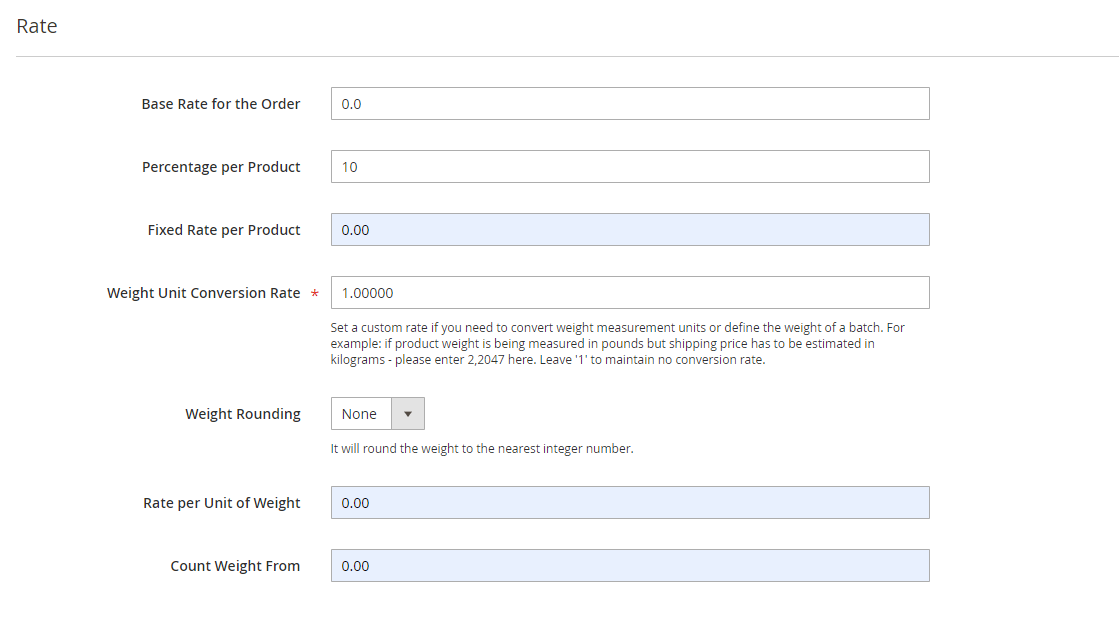Screenshot of an Order Configuration/Rate Menu:
 
- **Appearance:** The background is entirely white.
- **Header (Top Left):** "Rate" indicated.

**Input Fields:**
1. **Base Rate for the Order:** Currently set at 0.0.
2. **Percentage per Product:** Currently set at 10.
3. **Fixed Rate per Product:** Currently set at 0.00 (displayed with a blue background).
4. **Weight Unit Conversion Rate:** Currently set at 1.00005. Includes a detailed note:
   - "Set a custom rate if you need to convert weight measured units or define the weight of a batch. For example, if product weight is being measured in pounds, but shipping price has to be estimated in kilograms, please enter 2.2047 here. Leave at 1 to maintain no conversion rate."
   - Marked with a red star, indicating it is required.
5. **Weight Rounding:** Currently set to "None," with a note:
   - "It will round the weight to the nearest integral number."
6. **Rate per Unit of Weight:** Currently set at 0.00 (displayed with a blue background).
7. **Count Weight From:** Currently set at 0.00 (displayed with a blue background).

All input fields have white backgrounds except for "Fixed Rate per Product," "Rate per Unit of Weight," and "Count Weight From," which have blue backgrounds.